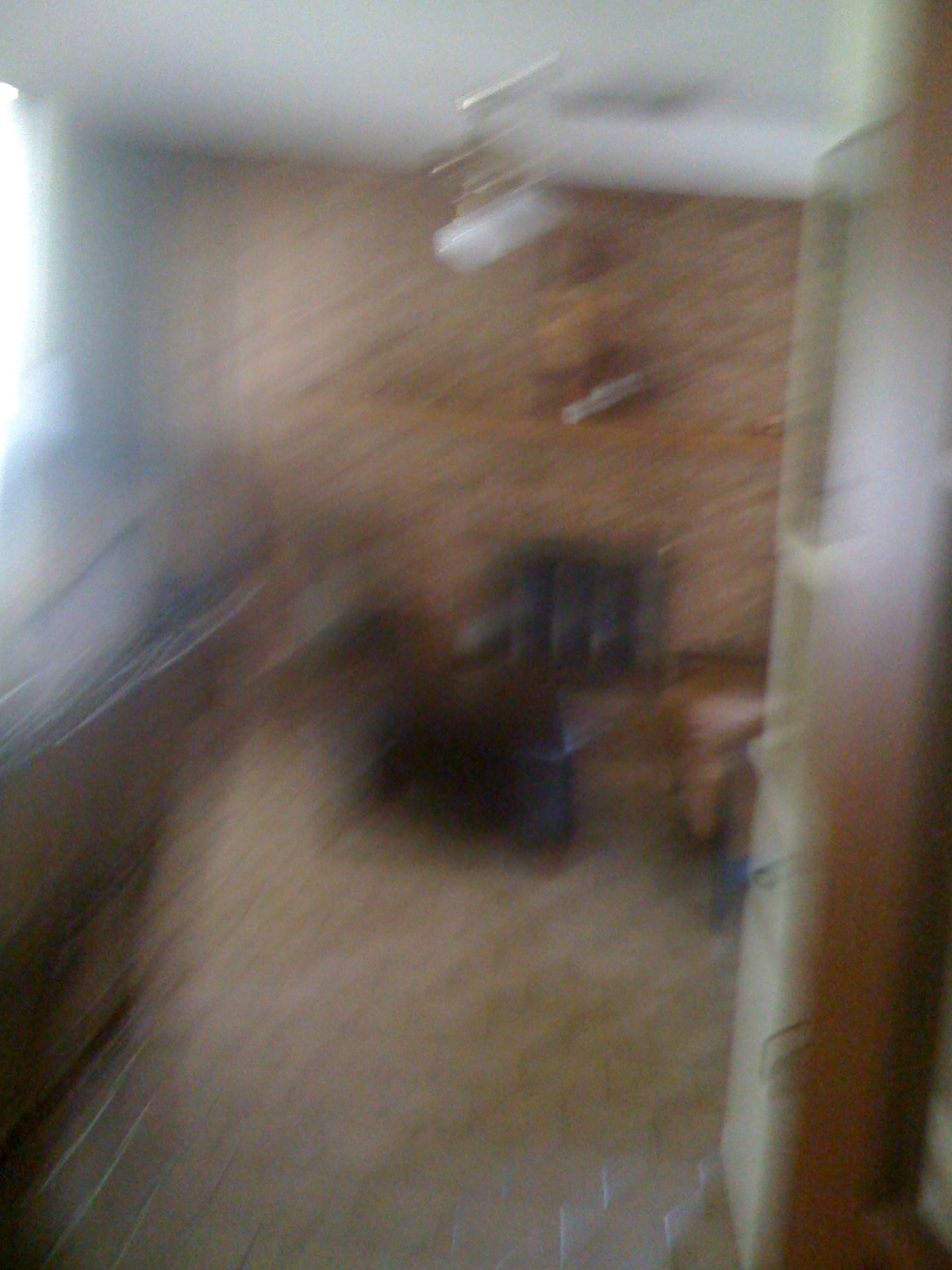**Descriptive Caption:**

In this blurred indoor photograph, a cozy living area is depicted with a warm, inviting ambiance. Central to the image is a brick wall, featuring a fireplace with a wooden mantel above it. On the mantel, though indistinct, there appears to be a portrait of a person wearing a brown hat, a yellowish face, and a brown jacket. 

To the right of the fireplace stands a wooden bookshelf with an off-white or birch interior. The bookshelf has two visible shelves and a pull-out drawer, with a cabinet underneath for additional storage. 

On the left side, partly obscured by the blur, there is a window possibly adjacent to a bar or another sofa, contributing to the layered, homely feel of the space. A black chair and a brown sofa furnish the room, adding to its cozy and lived-in atmosphere.